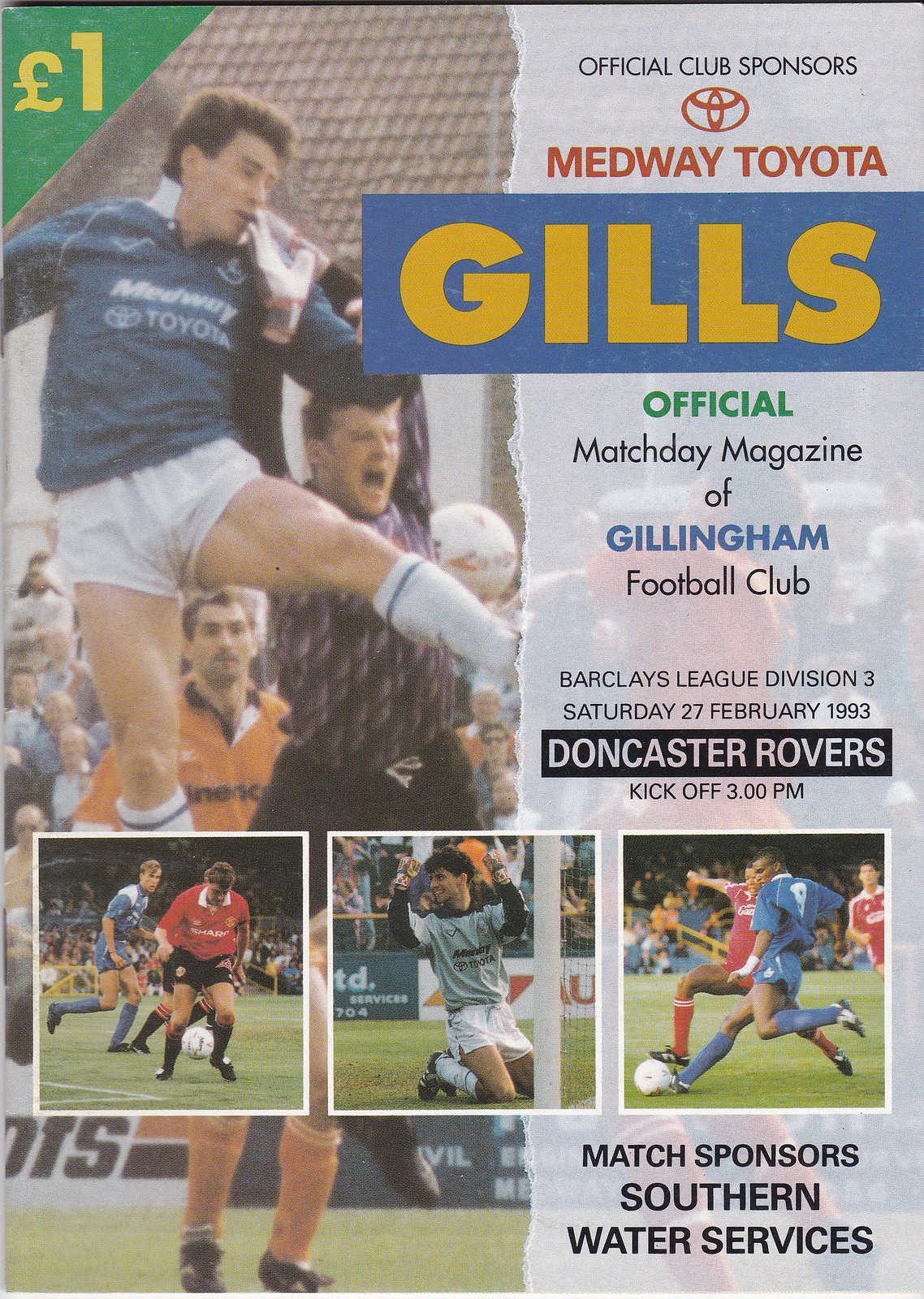This detailed football match program flyer, from February 27, 1993, likely from a vintage event, captures the essence and excitement of the game. Dominating the top left corner is a green triangle with "One Pound" highlighted in yellow. To its right, "Official Club Sponsor" is prominently stated above an image of a Toyota, followed by "Medway Toyota" underneath.

Centered on the flyer is a dynamic photo of a soccer match featuring players in action: a footballer in blue tackling mid-air with an opponent in black, along with visible players in orange jerseys and an engaged crowd in the stands. Just below, the headline "GILLS" is displayed in bold, capitalized letters within a blue rectangle with vivid yellow text. Further down, information about the match reads: "Official Match Day Magazine of Gillingham Football Club, Barclays League Division 3, Saturday, 27 February 1993, Doncaster Rovers, Kick-off 3 p.m."

At the bottom section, three smaller images showcase various moments of the game: the first depicts three players, one in blue and two in red, engaged in play; the center image captures a goalkeeper in action, kneeling with raised hands; the third image features a player in blue and two in red competing for the ball, with the audience and sponsor banners in the background.

Concluding the flyer on the bottom right is "Match Sponsors: Southern Water Services," rounding out the visual and textual elements that celebrate this eventful football match.